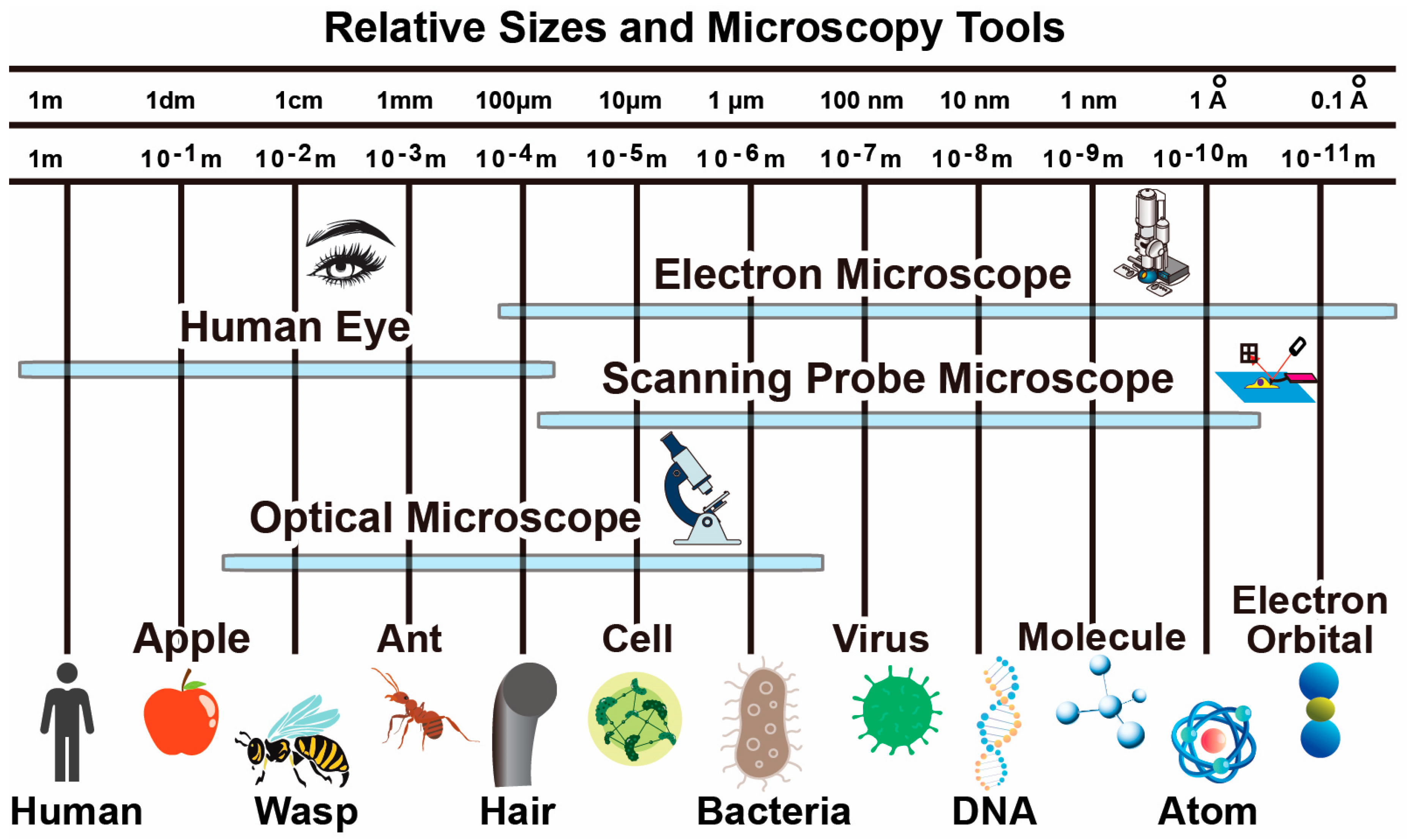This is a detailed color diagram illustrating the relative sizes of various objects and the microscopy tools used to observe them. At the top, the scale spans from 1 meter (1M) on the left to 0.1 angstroms (Å) on the far right, covering a range of measurements: 1 decimeter (1DM), 1 centimeter (1CM), 1 millimeter (1MM), 100 micrometers (100µm), 10 micrometers (10µm), 1 micrometer (1µm), 100 nanometers (100nm), 10 nanometers (10nm), 1 nanometer (1nm), down to sub-nanometer scale. 

From left to right, the diagram depicts progressively smaller entities starting with a human (visible to the naked eye), followed by an apple, a wasp, an ant, a human hair, a cell, bacteria, a virus, DNA, molecules, atoms, and finally electron orbitals. Each object is accompanied by minimalist, colored cartoon drawings and labels. 

Above and below the scale are indicators of the observational tools suited for each size range. The human eye can see objects down to about 100 micrometers, which includes items like a human, an apple, a wasp, and an ant. The optical microscope extends the visible range further to include structures like hair, cells, and some bacteria. To view entities like viruses, DNA, and smaller molecules, electron microscopes or scanning probe microscopes are required. The smallest depicted structures, such as atoms and electron orbitals, require the high resolution of electron microscopes.

Blue rectangular lines beneath the illustrations demarcate the range of visibility for each tool, including the human eye, optical microscope, scanning probe microscope, and electron microscope. This comprehensive layout effectively communicates the scale of various objects and the corresponding microscopy tools necessary to observe them.